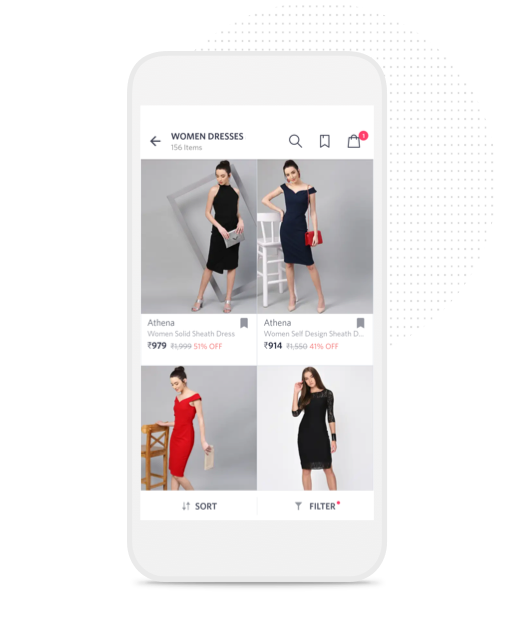This image is a screenshot taken from a smartphone, which is depicted with a cartoonish outline in a generic pale gray color, devoid of any branding. The smartphone's screen shows a website displaying four images of women modeling dresses. These images are arranged in a 2x2 grid, with three of the dresses in black and one, located in the bottom left, in a striking red. The models, all brunettes with their hair pulled back, except for the model in the bottom right image who has long, flowing brown hair, pose against a gray backdrop. The backdrop varies slightly in shade, with three of the images featuring a dark gray background and the bottom right image featuring a lighter, pale gray background. Surrounding the smartphone screen are numerous gray dots aligned in horizontal rows, forming a circular shape, adding an additional graphical element to the overall design of the screenshot.